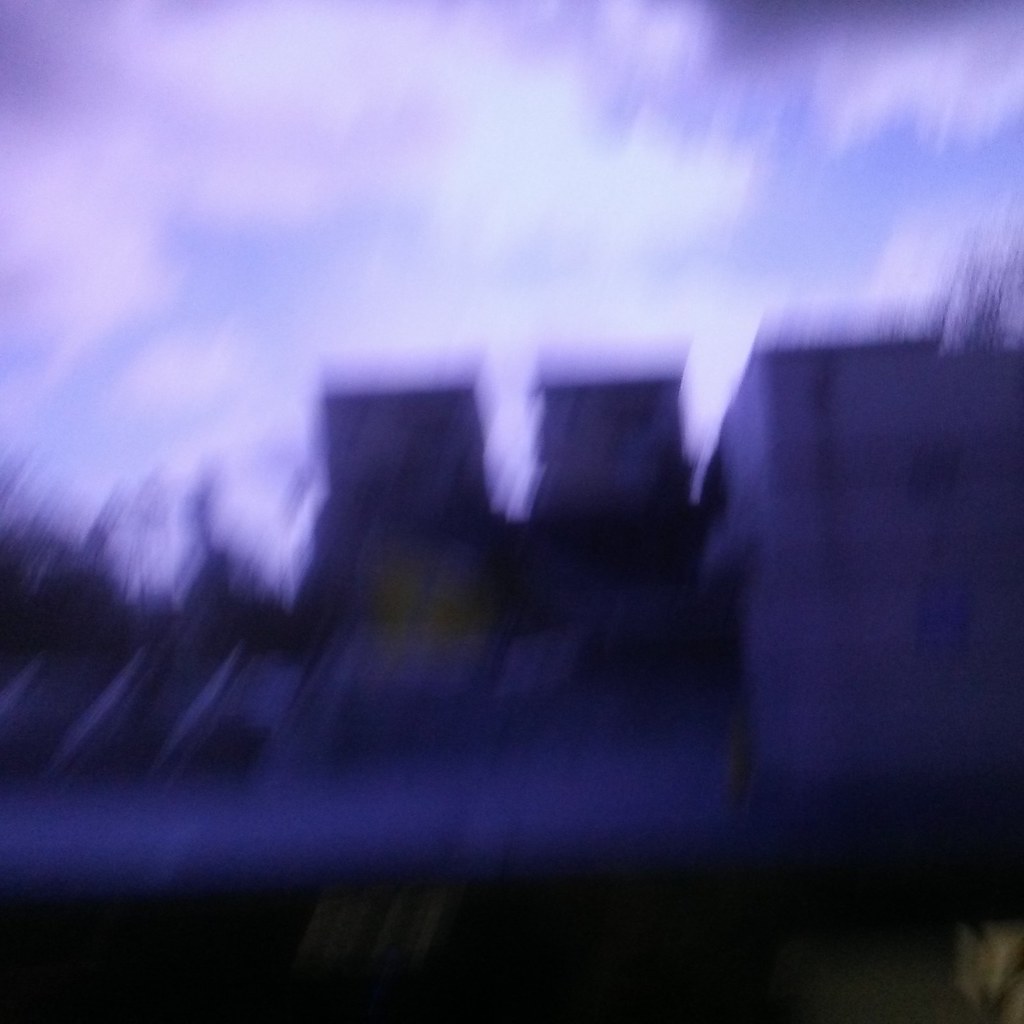The image captures an outdoor scene during twilight, characterized by a dark purplish-black ambiance. In the foreground, there is a square white object, flanked by two tall, square structures on its left. Adjacent to these structures are three white dashes, followed by a black line with white vertical lines running through it at the bottom. The background reveals a landscape of dead trees, which appear grayish-black, adding to the somber mood. The sky above is a mix of ominous clouds, softly illuminated by the remnants of sunlight. In the bottom right corner, a green plant provides a contrasting pop of color against the darker hues.